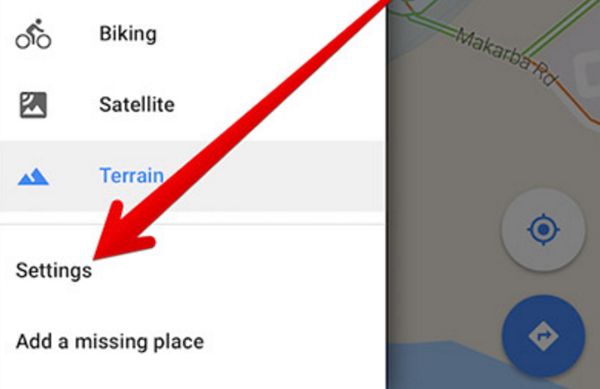In this zoomed-in image of a website, the focus is on the left panel featuring three distinct logos and related descriptions. The first logo depicts a person on a bicycle with two wheels, representing "biking." The second logo showcases a mountain with a small satellite at the peak, symbolizing "satellite." The third logo features a blue terrain mountain, labeled as "terrain." Next to these logos, there are three corresponding icons with descriptive tags: "biking," "satellite," and "terrain." Below these elements, there are options for "settings" and "adding a missing place."

On the right side of the image is a grayed-out, rectangular map, marked prominently by a large, downward-pointing arrow directing attention towards the "settings" option. The background of this interface is white, with the text for "terrain" standing out in blue. Additionally, the map section includes a visible road labeled "Maka'arba Road." Just below the map, there are two small buttons; one featuring a crosshair icon with a circle inside, and another blue button with a right-pointing arrow.